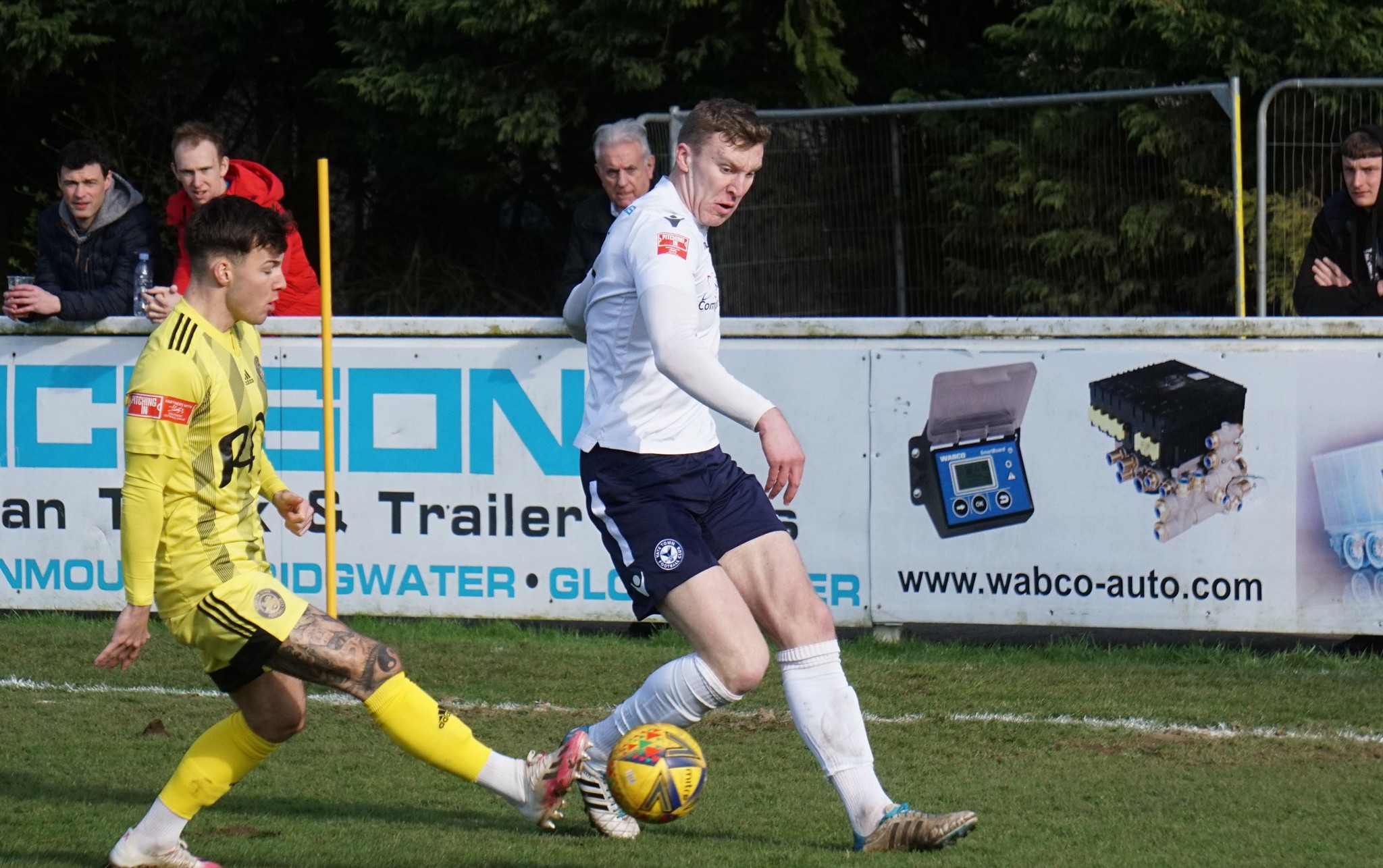This vibrant outdoor soccer match photo showcases two players in the midst of a heated battle for possession of a yellow soccer ball. The player on the left is dressed head-to-toe in yellow with black accents and sports tattoos on his leg. He is poised to kick the ball. His opponent, dressed in a white shirt, white knee-high socks, and dark blue shorts, displays a comical yet intense expression as he tries to intercept. The green soccer field behind them is clearly marked. In the background, several spectators—two men in blue and red jackets, another in a black hoodie, and a partially visible older man with silver hair—are watching eagerly from behind a white wall adorned with advertisements. The ads feature text about "sun, trailer, something, water," pictures of electronic devices, and the website www.wabco-auto.com. Surrounding the scene, abundant greenery, including trees and shrubs, creates a lush backdrop. The array of colors, including black, white, red, green, yellow, various shades of blue, brown, and gray, enhance the image's vivid detail.